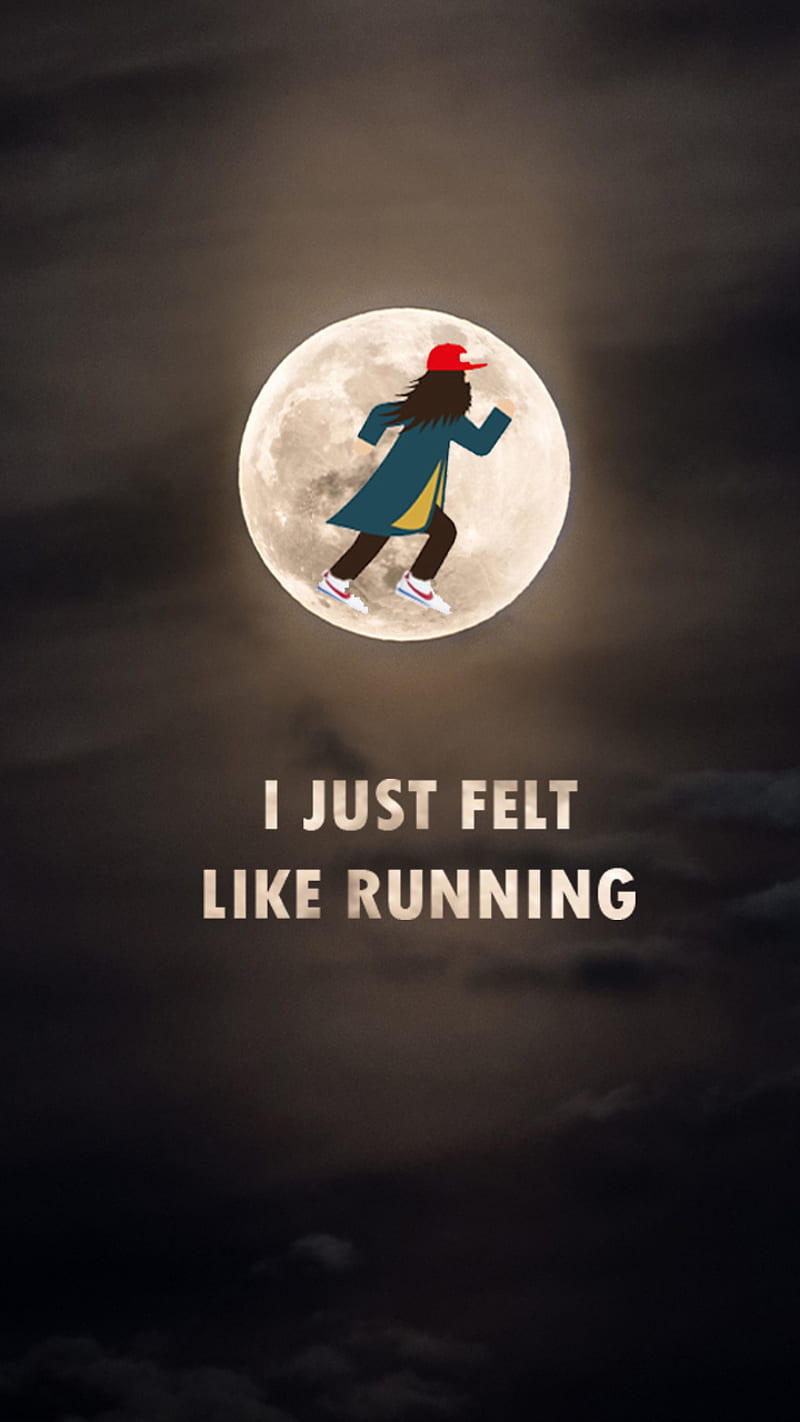This digital art piece, inspired by the movie "Forrest Gump," features a vertical rectangular composition. The background depicts a night sky with clouds, with the moon positioned in the upper middle portion. The moon casts a soft glow that subtly suggests moonlight filtering through thin, wispy clouds. Prominently, a comic book-style illustration of Forrest Gump is depicted running across the moon from left to right. 

He wears a red baseball cap and has long, full hair and a beard. His attire includes a blue and yellow jacket, brown or dark pants, and iconic white Nike running shoes with red stripes. Below the moon, in bold white letters, the text reads, "I just felt like running," capturing the essence of the character's memorable quote from the film. The overall color palette includes shades of black, brown, and beige, enhancing the nighttime ambiance of the scene.